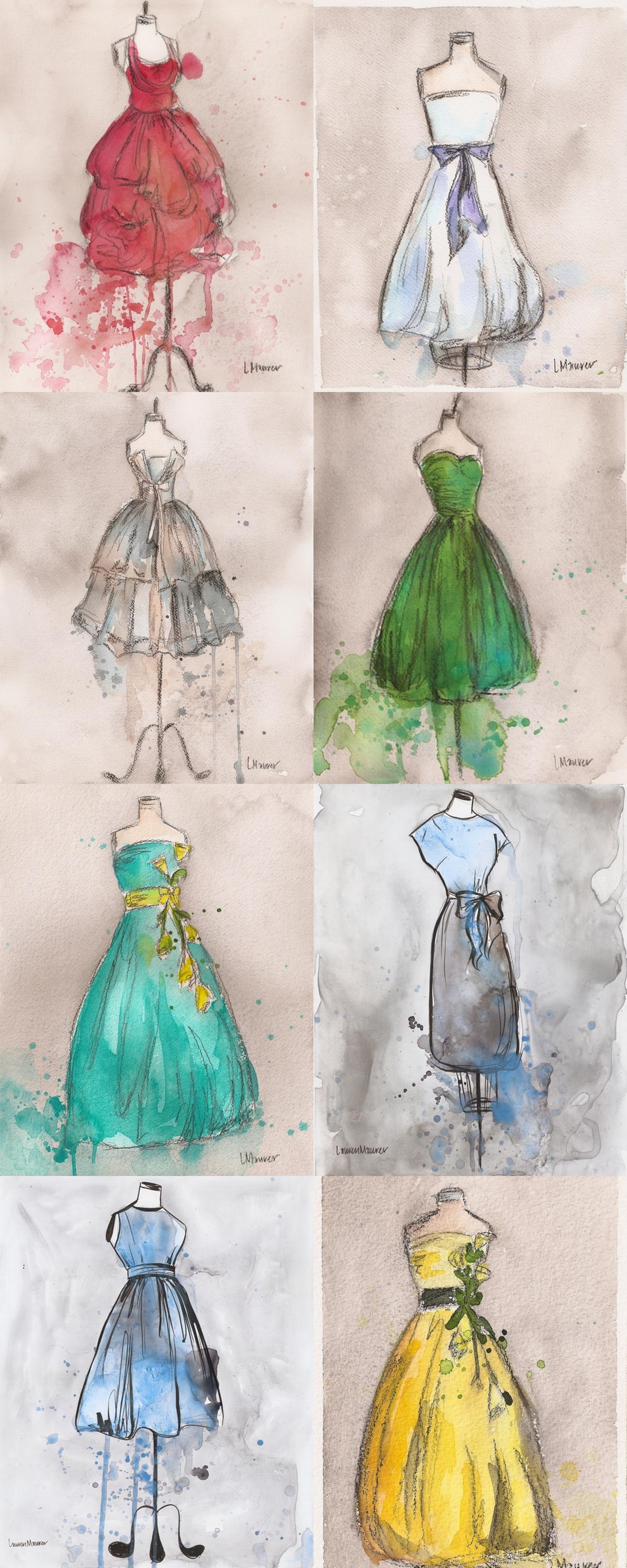The image showcases a fashion illustration featuring eight watercolored dresses arranged in two columns against a cloudy gray and white background. Starting from the left column, the top dress is a short, sleeveless red dress. Below it is a white sleeveless dress accented with a purple bow around the waist. The next dress down is a short, sleeveless gray dress with a roughly textured appearance. At the bottom of this column is a turquoise-colored gown with a yellow sash adorned with flowers.

In the right column, the top dress is a white sleeveless dress with a purple bow around the waist, mirroring the one mentioned previously. Below it is a deep green, short, sleeveless dress with a fitted bodice. The next outfit is a modern ensemble featuring a light blue top paired with a gray pencil skirt and a gray bow. The final piece in this column is a longer, sleeveless yellow gown with a black sash around the waist, complemented by floral detailing.